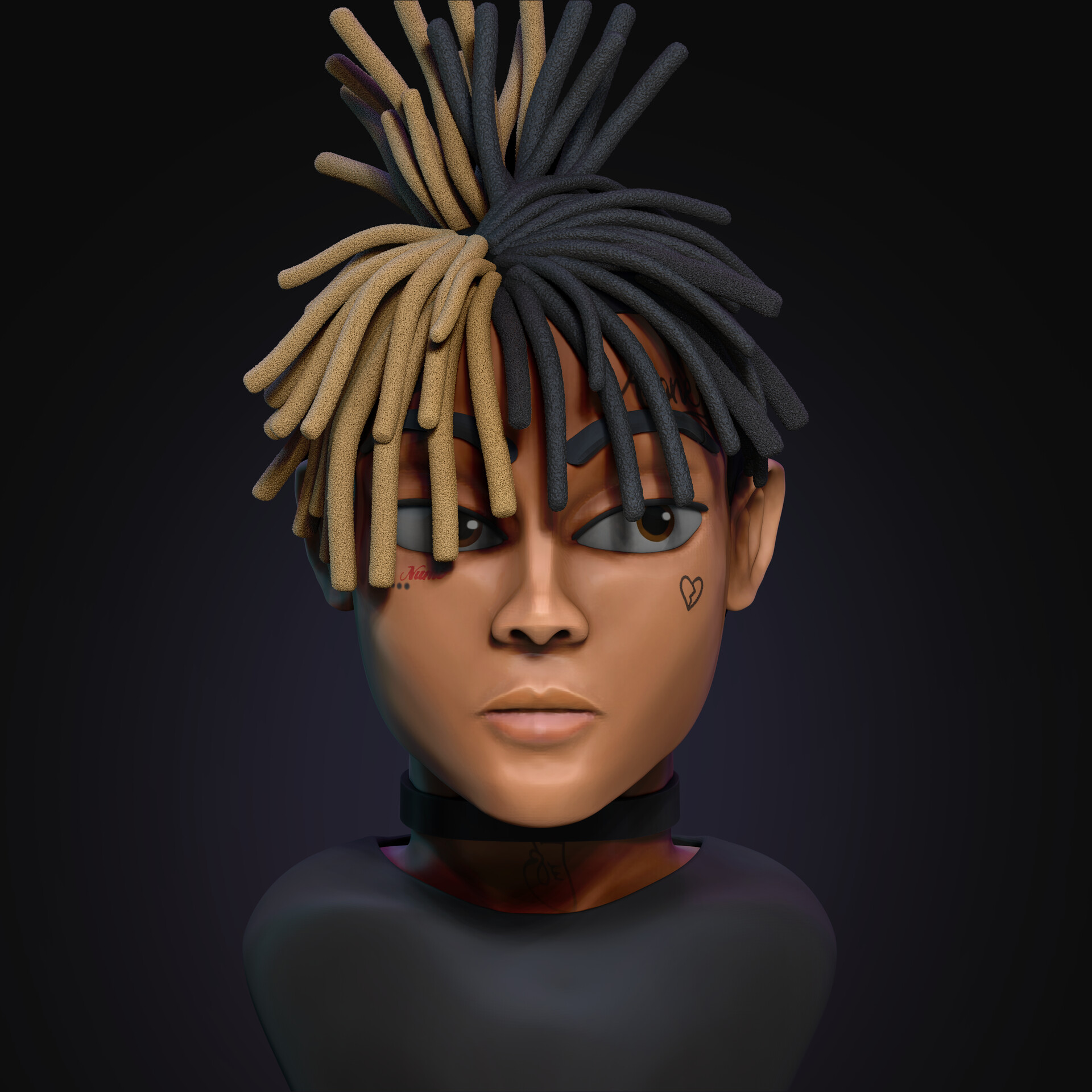The image is a stylized, abstract representation of a person's head and shoulders depicted against a black background. The figure's hair is divided into thick, spaghetti-like dreadlocks, with the left side being light brown and the right side black. The person's face features exaggerated, oversized eyes and eyebrows, giving it a cartoon-like quality, yet maintaining some human-like characteristics. A heart tattoo is situated below the left eye on the figure's cheek, and another smaller tattoo, appearing to consist of letters and dots, is found beneath the other eye. The individual is depicted without visible arms, the shoulders being truncated, reminiscent of a mannequin. The neck is adorned with what seems to be a tight, dark-colored band or high-collared shirt, matching the dark tones of the hair. The figure is gazing to their left, adding to the overall enigmatic and artificial aesthetic, enhanced by the smooth texture of the skin.